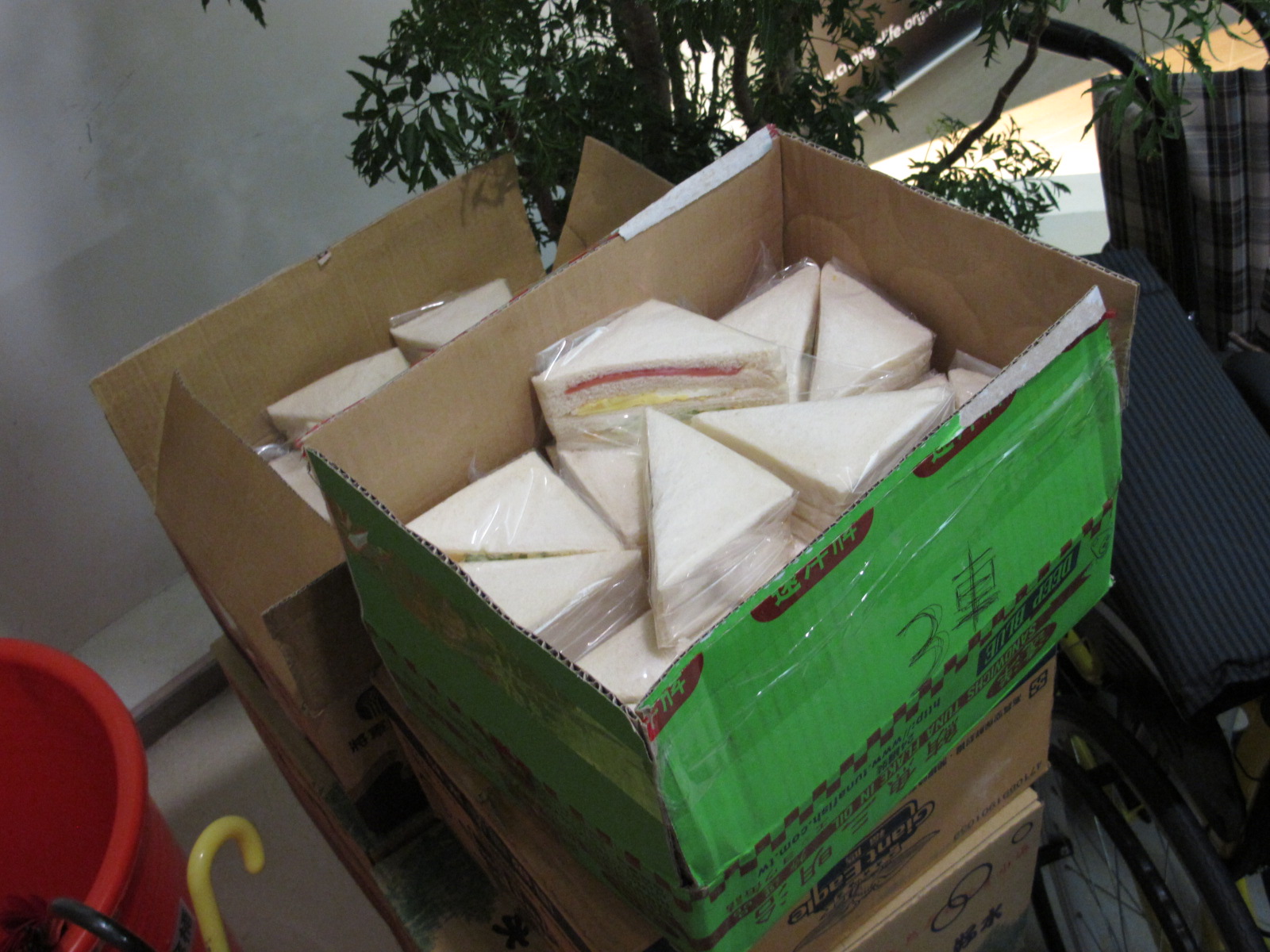This detailed photograph shows a stack of sandwiches made with white bread, cut into triangles and wrapped neatly in clear plastic. These sandwiches, featuring a pinkish-red filling and a layer of yellow and white filling, are piled up within a series of boxes. The topmost box, which is green and adorned with Asian lettering, is open, revealing the neatly stacked sandwich halves inside. Below and behind this green box are several brown cardboard boxes, possibly containing more sandwiches. 

To the right of these boxes stands a manual wheelchair with a plaid backrest, positioned next to a house plant with several thick stems. The scene is lit by sunlight streaming through a window behind the plant. Additional details include a red bucket with a piece of yellow plastic, curved like a candy cane, in the lower left-hand corner of the image. The wall in the background is white, and the overall setting appears to be indoors, possibly near an office or residential area with a welcoming and orderly atmosphere.